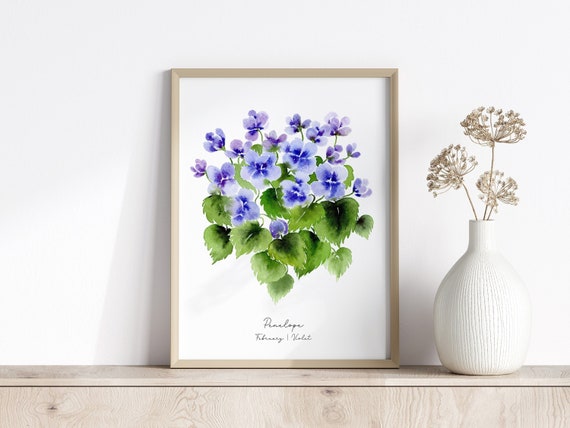The photograph depicts a serene indoor setting featuring a light brown wooden shelf. Centrally positioned on the shelf is a painting bordered by a thin, light brown frame. The artwork showcases vivid green leaves and blueish-purple flowers, identified as violets, along with an indistinguishable signature that includes the word "violet." To the right of the painting sits a white vase, adorned with textured lines, containing three brown flowers. The backdrop is a pristine white wall, complementing the overall elegant and tranquil ambiance. The colors in the scene span various shades, from the blue and lavender hues of the flowers to the greens of the leaves, and the browns of the shelf and frame. This composition, likely situated in a cozy home, brings a touch of nature indoors.